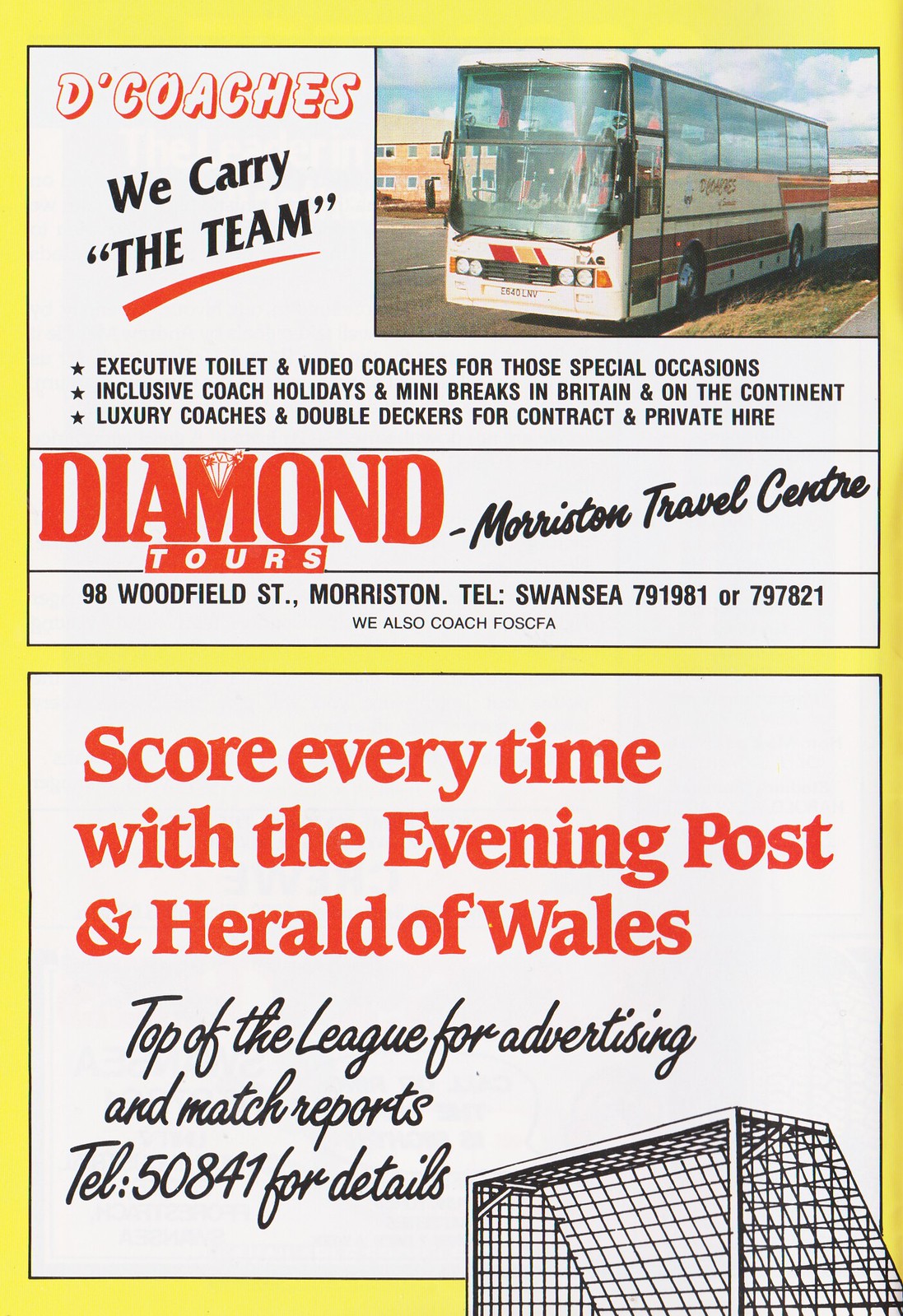The image is a page out of an old magazine with a yellow background, divided into two sections with advertisements. The top section features an ad for Diamond Tours, containing a coach bus image in the top right corner. The ad details various services including executive, toilet, and video coaches for special occasions, inclusive coach holidays, and mini breaks in Britain and the continent. It also mentions luxury and double-decker coaches for contract and private hire, with contact details for Morriston Travel Center. The bottom section is an advertisement for the Evening Post and Herald of Wales, promoting their superiority in advertising and match reports with the slogan "Score every time," displayed in red text on a white background. The phone number for more details is also provided. Together, these well-spaced advertisements evoke the vintage style of the magazine page.